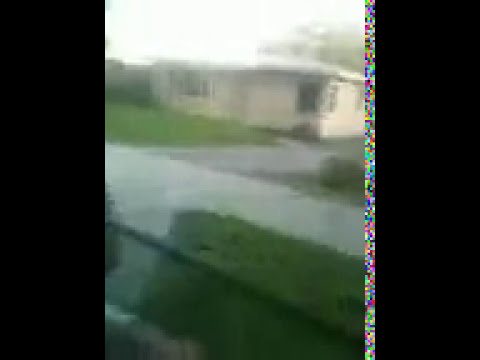The image is a very blurry, low-quality photograph of a small, one-story house with a gabled roof, predominantly light cream or beige in color. The photo, seemingly taken from inside a car, depicts a driveway of dark gray asphalt on the right side and a concrete sidewalk stretching from the bottom right to the upper left, separating the house from a green lawn. The roof appears flat due to the haziness, with sunlight glaring off it, which obscures the sky above. A large green tree is visible above the house on the right, and on the house's right side, there are two dark, nearly black windows. An additional window, also dark, is situated in the right corner of the house, and a porch with a dark square at its center is seen on the left. The right side of the image features vertical pixel artifacting in a multicolored band, indicating digital distortion. The photo is the middle panel of a triptych, bordered by black panels on either side, with a multicolored border running between the center and right panel. In front of the house, on the other side of the sidewalk, lies a thick, large green shrub.